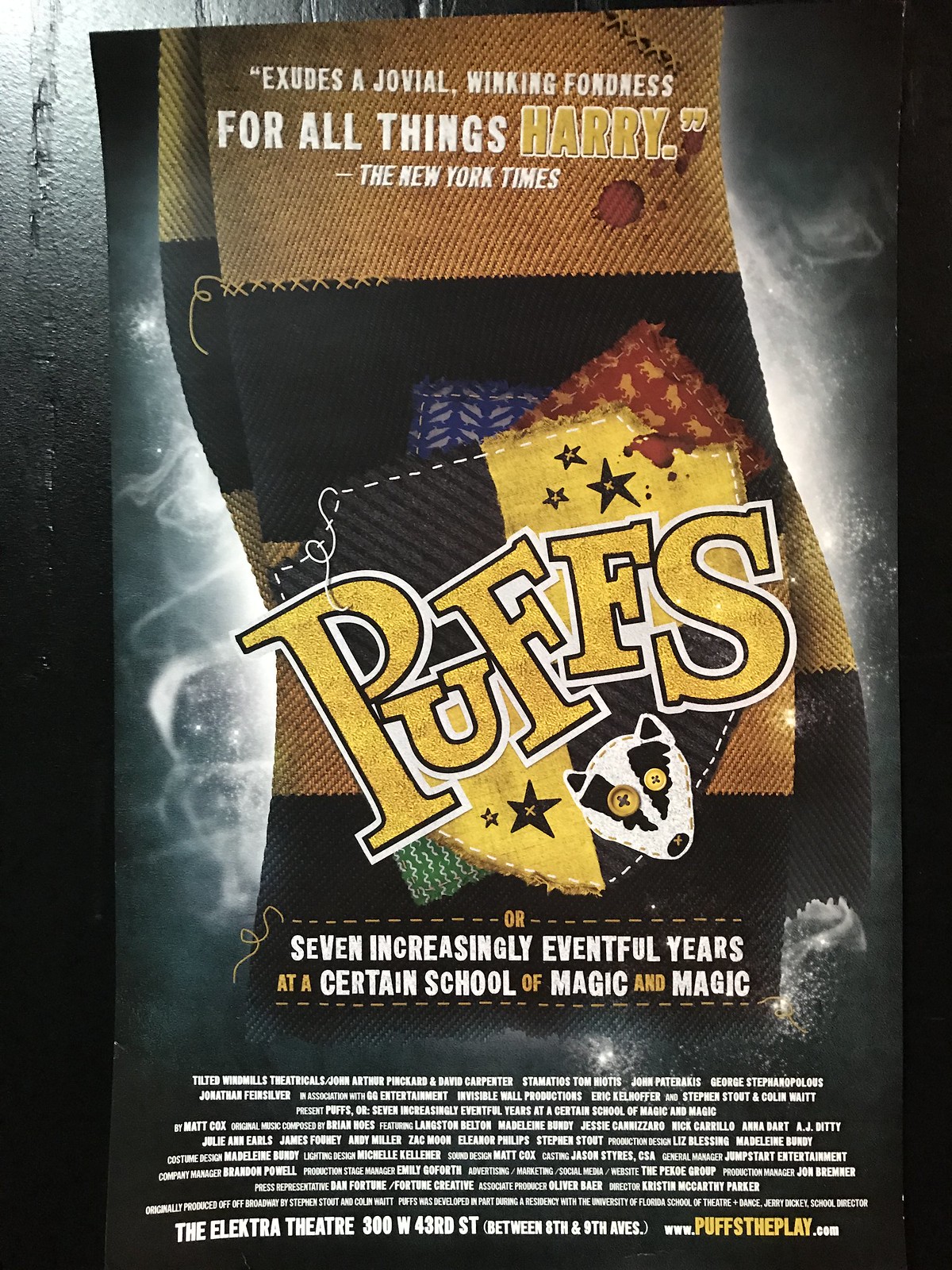The image is a detailed promotional poster for a theater production titled "Puffs." The poster, which is rectangular and taller than it is wide, has a background consisting of a black and gray smoky design that gives the appearance of a wall. A central element is a yellow and black striped scarf, over which a fabric shield logo is displayed. The shield is quartered with yellow and black sections, adorned with stars, and a badger's head beneath the two "F"s in "Puffs."

At the top of the poster, white text reads: "Exudes a jovial winking fondness for all things Harry – The New York Times." Below this, in the center, the title "Puffs" is prominently written in a yellow font with a white border. Below the title, additional text in white and gold reads: "Seven increasingly eventful years at a certain school of magic and magic."

Towards the bottom, the poster includes smaller text that is mostly illegible, ending with a readable address: "The Electra Theater, 300 W 43rd Street, between 8th and 9th Avenues." The bottom-right corner displays the website: "www.puffstheplay.com" with "Puffs the Play" in gold font.